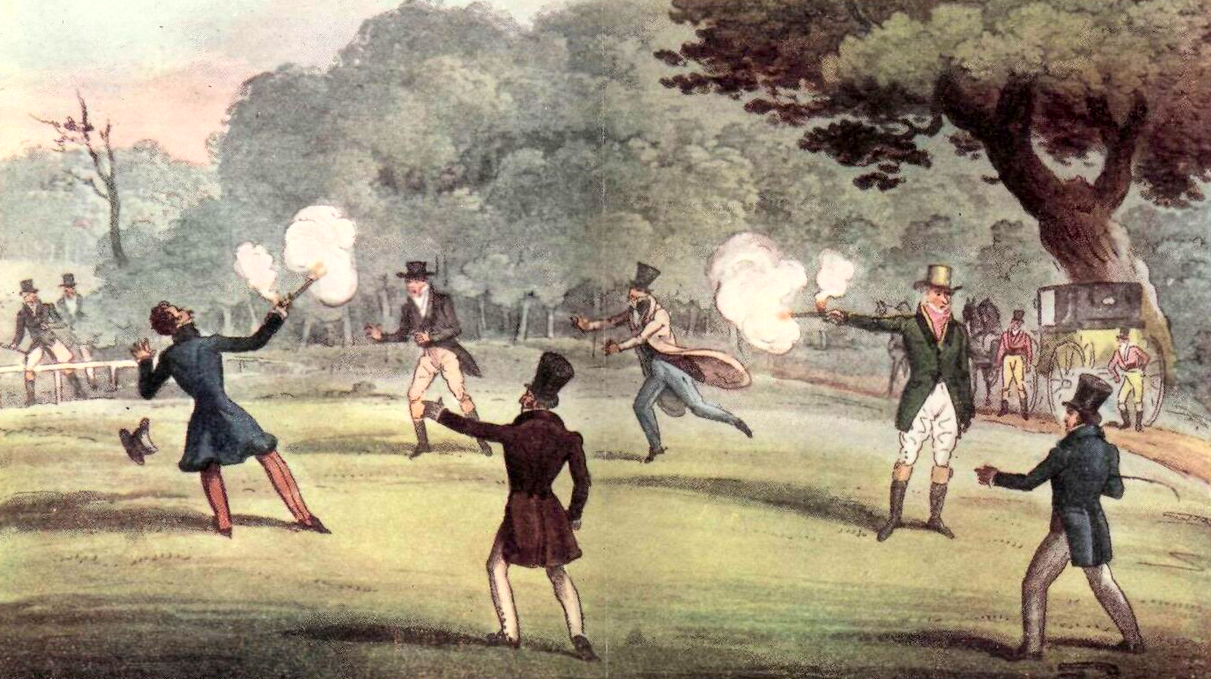The image depicts a detailed, color painting set in what appears to be a park during the Civil War era. Central to the scene are two men engaged in a dramatic shootout, each discharging Civil War-era pistols with billowing clouds of white smoke. The man on the left, dressed in a green jacket and white trousers, aims his pistol at another man to the right, who is tilting backward with smoke issuing from his gun, suggesting he has been shot. This second man, distinguished by his lack of a hat—perhaps knocked off in the skirmish—is falling to the ground.

The background features a dense, green park-like area with trees visible and a horse-drawn carriage stationed on the left. Spectators in old-fashioned clothing, including elegant suits and top hats, are scattered across the scene. On the right side, a group of onlookers in red jackets and yellow trousers, possibly soldiers, are either running for help or simply observing the chaos. The scene is meticulously detailed, capturing not just the central conflict but also the surrounding elements, providing a vivid snapshot of a bygone era.